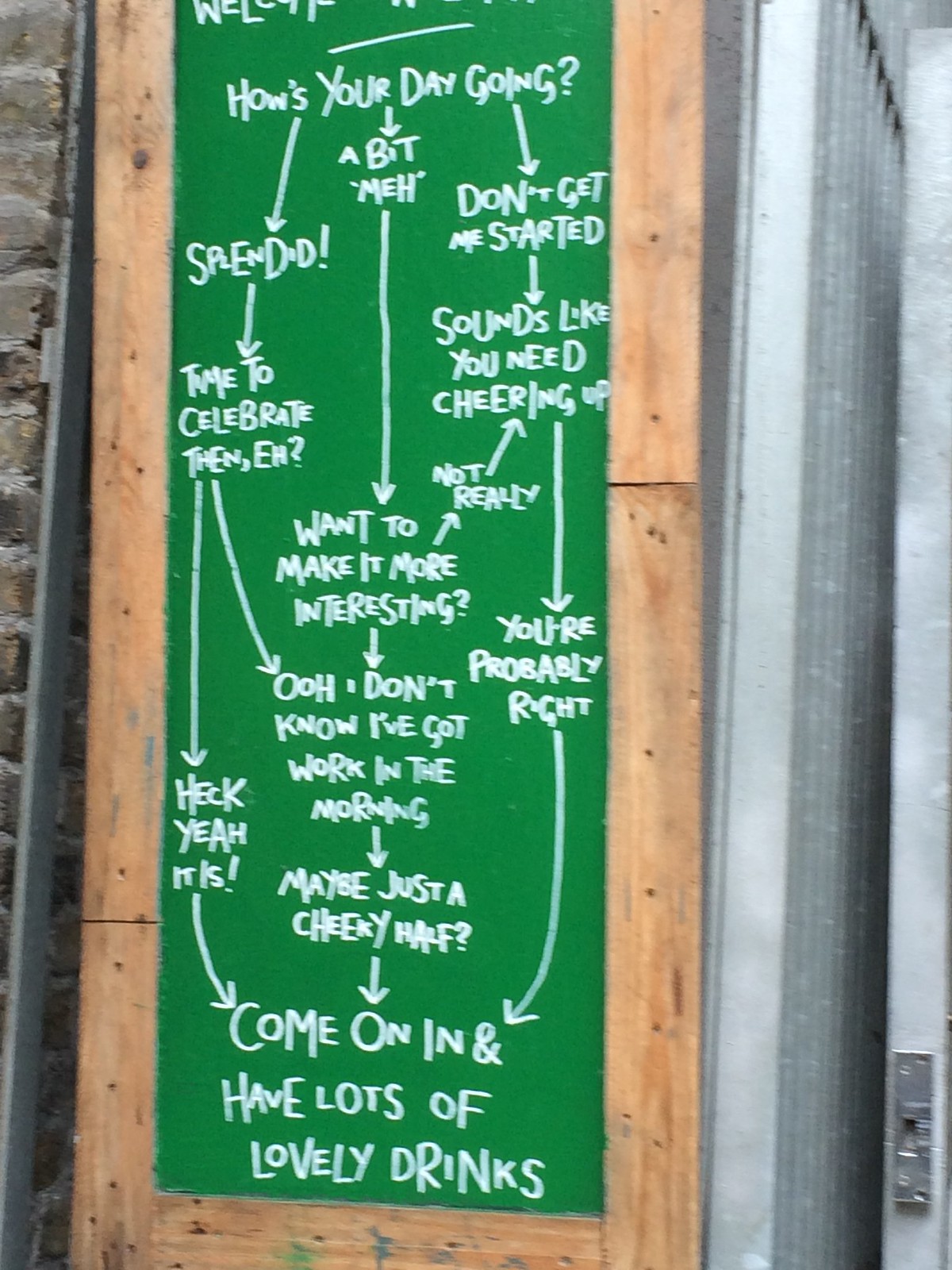This vertical rectangular photograph captures a green chalkboard sign, framed in rough, bare wood, mounted on the exterior brick wall of what presumes to be a bar. The sign, detailed with whimsical white chalk writing, serves as an engaging flowchart starting with the question, "How is your day going?" 

Arrows guide the viewer through three primary responses: "Splendid," "A bit meh," and "Don't get me started." Each path humorously converges towards the inviting suggestion to "Come on in and have lots of lovely drinks." 

One path reads: "Splendid -> Time to celebrate, then, eh? -> Heck yeah, it is!" Another path follows: "A bit meh -> Want to make it more interesting? -> Oh… don't, no, I've got work in the morning -> Maybe just a cheeky half?" The final path: "Don't get me started -> Sounds like you need cheering up -> You're probably right."

This evocative and playful sign not only serves as charming decor but also creatively entices visitors to step inside for a drink, promising a respite regardless of how one's day is going.